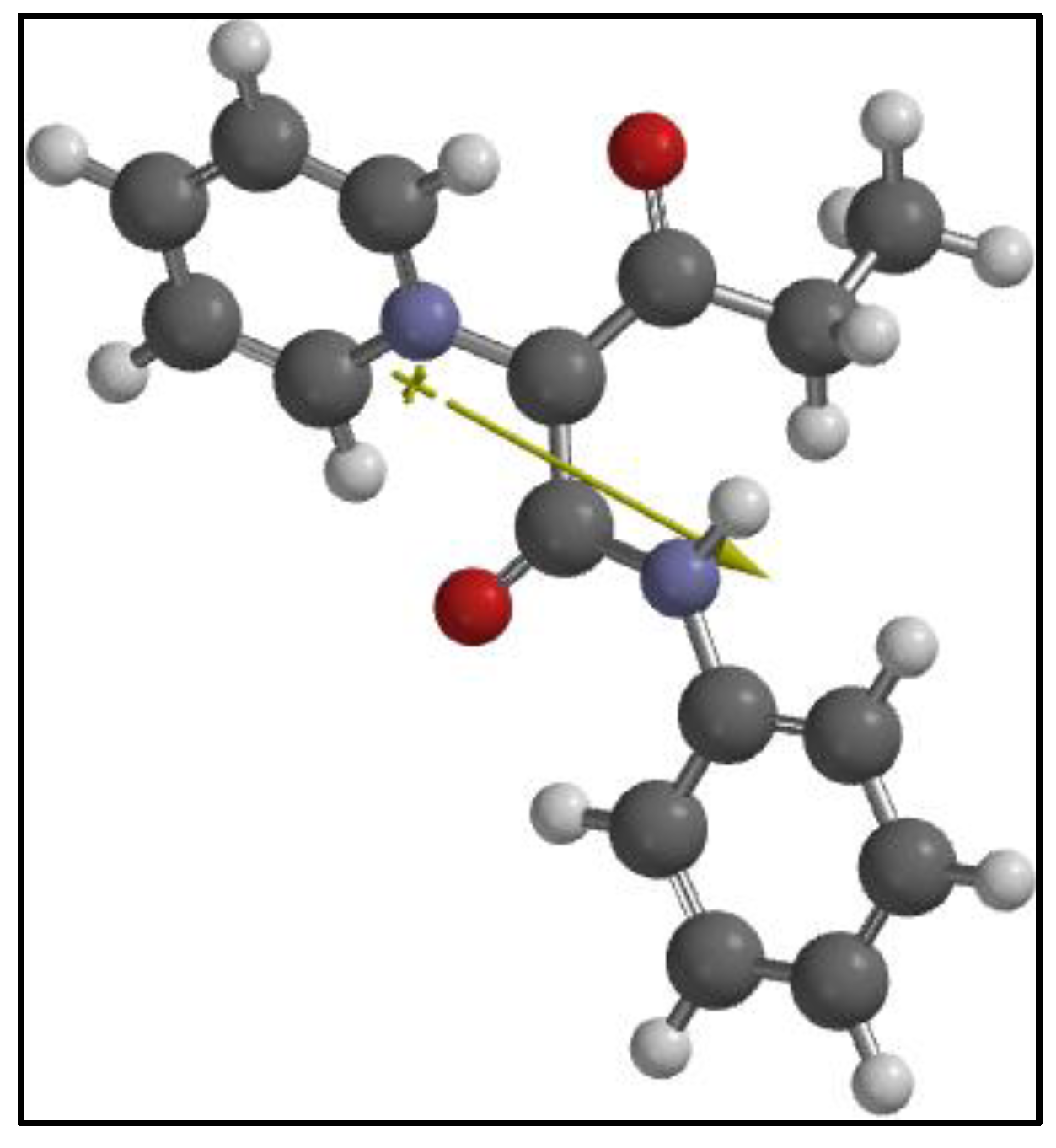The image vividly depicts a complex molecular structure, consisting of various colorful molecules interconnected by silver spokes. Beginning at the upper left corner, smaller outer molecules are light gray, linked by stems to larger, darker gray circles. As the structure progresses toward the right and downwards, different molecules including blue, red, and a unique light green cross shape are observed. Among the mix, a couple of molecules are also light purple. A prominent yellow arrow is drawn diagonally from the middle top of the image, guiding from left to right and downwards, highlighting the direction of the molecular sequence. The intricate network extends to touch the bottom right corner, contrasting with a vast expanse of white space occupying the bottom left quadrant of the image, enhancing the visual prominence of the molecular formation.